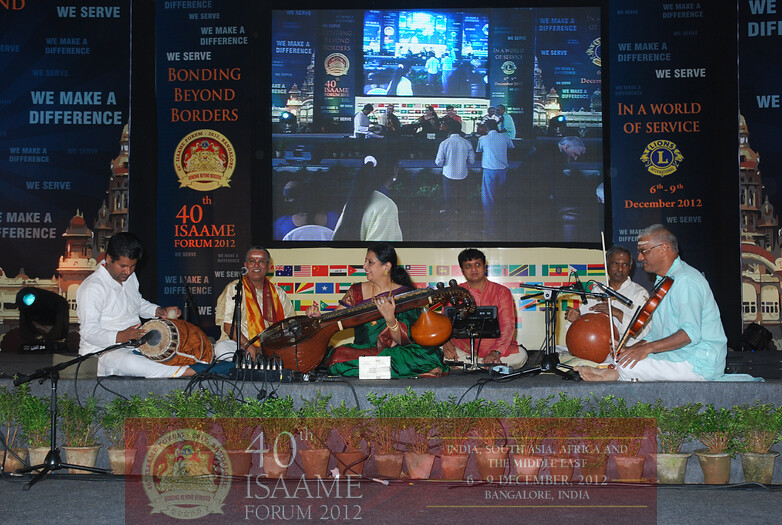In this image from the 40th ISAAME Forum 2012 held in Bangalore, India from December 6-9, 2012, a group of performers of Indian descent are seated at the center of a stage, playing various traditional Indian instruments. The stage, adorned with gray decor and terracotta pots with green plants, is likely set outdoors. A woman in the center holds a large, gourd-shaped string instrument while other musicians, including a man playing a cylindrical drum, a keyboardist, and two additional men, one with a round instrument and the other with a microphone, accompany her. Behind them is a large screen displaying their performance and the audience. The backdrop features black banners with text stating, "We make a difference. We serve bonding beyond borders." and "40th ISAAME Forum 2012." Along the bottom of the image is a transparent red rectangle with a gold seal on the left and white print reiterating the event details: "40th ISAAME Forum 2012, India, South Asia, Africa, and the Middle East, 6-9 December 2012, Bangalore, India."